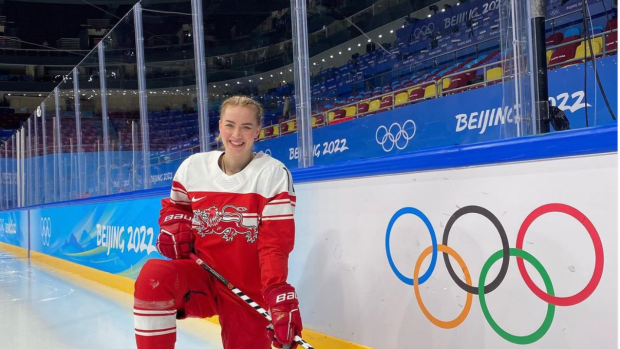The image captures a smiling blonde, white female hockey player, wearing a red jersey with a white upper section, kneeling on the ice of an ice hockey rink. Her red gloves, red pants, and red and white socks complement her outfit. The knee she is taking rests right next to the blue border wall emblazoned with "Beijing 2022" and the Olympic rings in white. The Nike logo and the letters "BAU" can be seen on her left gloves. She holds the upper part of her hockey stick with both hands, her pose illustrating a moment of pride and joy against the iconic backdrop. To her right, the five interlinked Olympic rings are vividly depicted in blue, yellow, black, green, and red against a white background. Behind her, the protective glass wall and further up, the stadium's empty blue seats are visible, indicating a quiet yet grand Olympic setting.